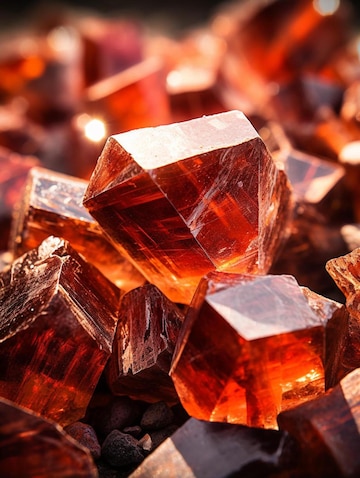This detailed image captures a close-up view of a random pile of deep red, blocky crystals, featuring flat surfaces and a transparent yet vividly colored appearance. The photograph's limited depth of field focuses sharply on four prominent crystals in the foreground, highlighting their large, irregular shapes and distinct edges. Some crystals display subtle yellow areas, adding complexity to their rich color. Though the precise type of crystal is uncertain, they evoke comparisons to amber or garnet due to their dark, ember-orange hue. The less polished arrangement suggests a natural clustering, possibly resting on wood chips or gravel. The background reveals many more crystals extending into a blurred distance, contributing to the scene's densely packed, textured composition.